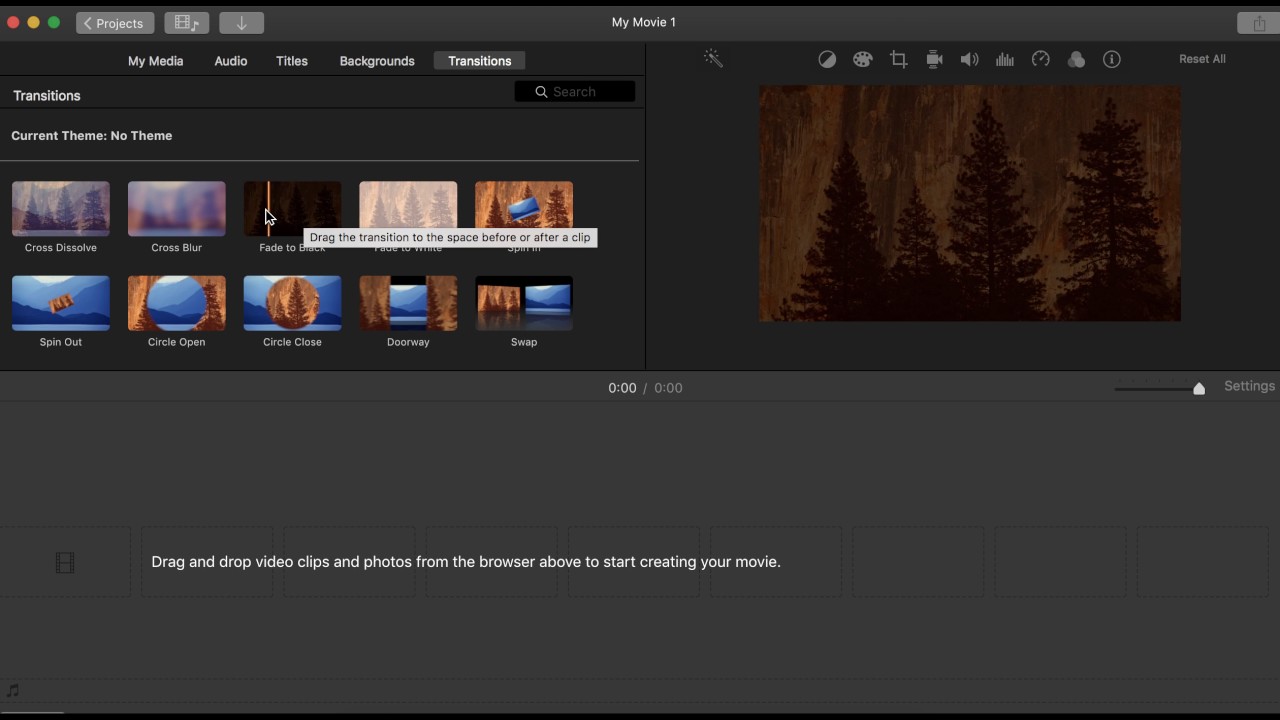Here's a detailed and cleaned-up caption for the image described:

---

A screenshot of video editing software is displayed, featuring a dark gray interface. Prominently across the top is the title "My Movie 1" in white text. In the upper left corner, there are three colored dots – red, yellow, and green – alongside a gray "Projects" button, a music icon, and a download arrow. 

The software's menus span horizontally across the top of the screen and include "Media," "Audio," "Titles," "Backgrounds," and "Transitions." The "Transitions" menu is currently selected, highlighted with small white text on a dark background. Directly below this menu, the phrase "Current Theme: No Theme" is visible in white.

The interface shows a selection of ten transition styles arrayed in two rows of five. Each transition icon includes a thumbnail preview and types such as "Cross Dissolve," "Cross Blur," and "Fade to Black." A tooltip is superimposed with the instruction, "Drag the transition to the space before or after a clip."

The second row of transition styles features options like "Spin Out," "Circle Open," "Circle Close," "Doorway," and "Swap." To the right of these transition options is an area displaying a template photo with a brownish-dark background and evergreen trees. Below this template, a text area instructs users to "Drag and drop video clips and photos from the browser above to start creating your movie," set against a clear gray background.

---